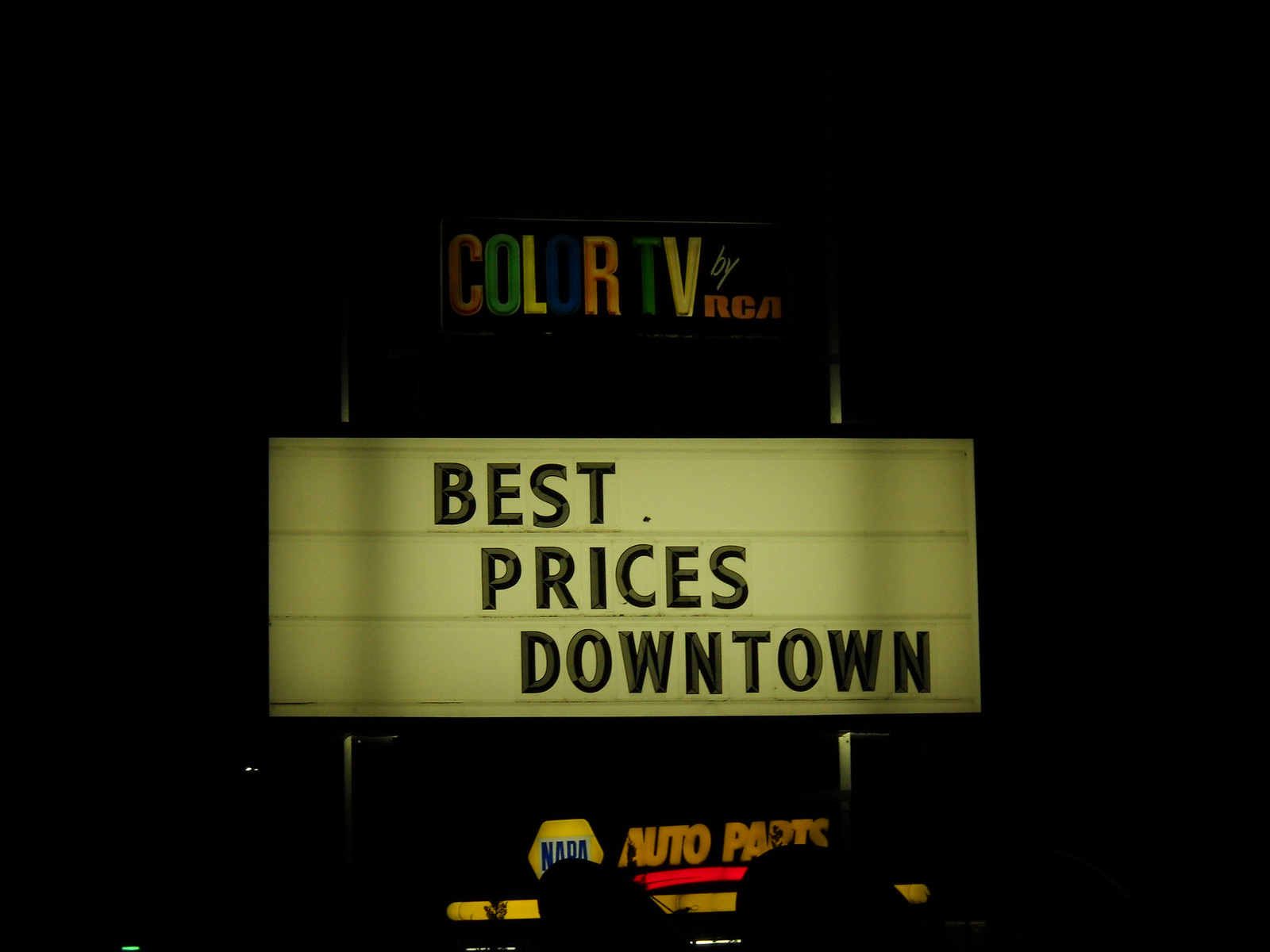This image, though poorly lit, prominently features a series of signs that provide the focal points of illumination. In the center, a partially lit white bulletin board-style sign with gray partition lines stands out. Bold black letters on this sign announce "Best Prices Downtown." Above it, a vibrant, multicolored sign with a black background advertises "Color TV by RCA" in red, green, yellow, blue, orange, and white letters. Below the white sign, another sign in striking hues of yellow, black, red, and hints of orange promotes "Napa Auto Parts." Despite the darkness surrounding them, these illuminated signs bring a vivid, almost nostalgic feel to the image.